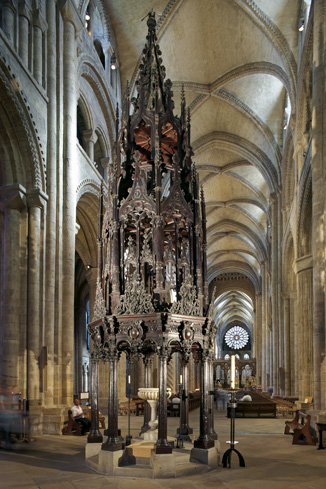The image captures the interior of an enormous cathedral, with intricate beige stone architecture. Majestic columns support towering archways, creating a sense of grandeur. Central to the scene is a large, aged statue, possibly bronze or gold, adding an element of historical elegance. At the far end, a stunning round stained-glass window in white and black features a beige center, casting a delicate light. Throughout the space, massive candlesticks with candles contribute to the cathedral's serene and hallowed atmosphere.